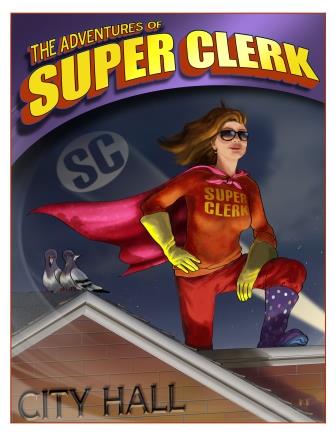The image features an advertisement or cover showcasing a female superhero in a striking red outfit complemented by a dark pink cloak and yellow gloves. She confidently stands atop a brown, sloping-roofed City Hall, striking a pose with one hand on her hip and the other resting on her knee or thigh. Her purple or blue boots and dark sunglasses add to her bold appearance, while her long, wavy dark brown hair flutters in the air. Two pigeons are perched on the city hall roof, which has a distinct triangular structure. The background features beacon letters "SC" illuminating the sky, symbolizing the superhero's alias, "Super Clerk." Prominently displayed at the top of the image in bold yellow block letters with a 3D red shadow, the title reads "The Adventures of Super Clerk," setting a dramatic and heroic tone for the character.